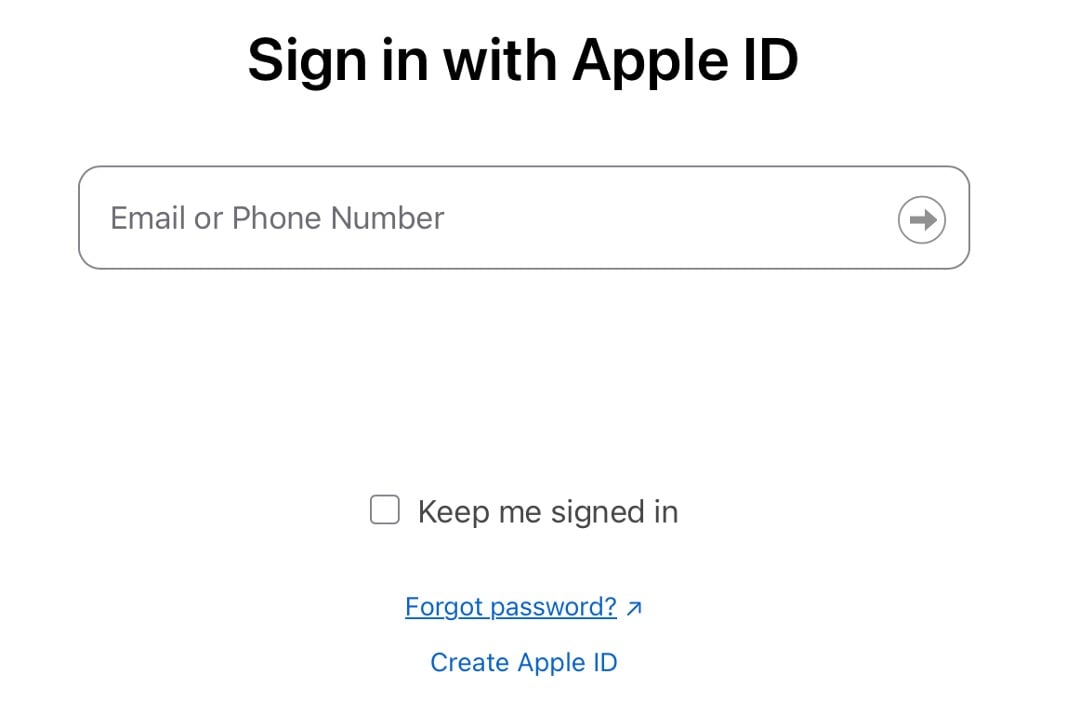The image displays the "Sign In with Apple ID" section, presented in large print centered prominently within the frame. No additional website elements are visible around this section. The text "Sign In with Apple ID" features capitalized letters: "S" in "Sign," "A" in "Apple," and both "I" and "D" in "ID." The remaining text is lowercase and well-spaced.

Beneath the main title, there is a clean, white rectangle with rounded edges, serving as an input field. Inside this field, the placeholder text reads "Email or Phone Number," where "Email" has a capital E, "Phone" has a capital P, and "Number" has a capital N. On the right side of this rectangle is a thick black arrow pointing to the right, contained within a circle.

Further down, the interface features another rounded rectangle that reads "Keep me signed in" on the right-hand side. Below this, there is a white space, followed by the text "Forgot password," which appears in blue font and is underlined with an arrow pointing to the upper right.

At the bottom of the section, the option to "Create Apple ID" is also displayed in blue font.